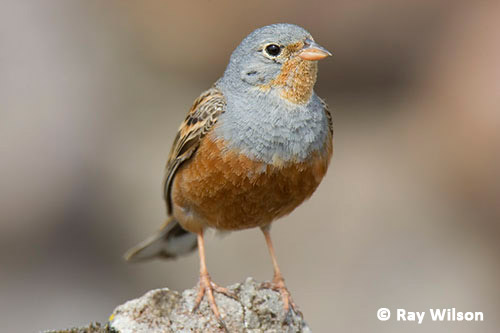In this detailed close-up image, a small bird stands prominently on a gray rock, surrounded by a blurry background that subtly transitions from gray to light brown. The bird features a striking light blue head and chest, gradually fading into a reddish-orange belly, with orange-tinted cheeks and forehead. Its beak is short and light orange, complementing the black eye positioned on the side of its head. The wings exhibit a pattern of black interspersed with brown and white feathers. Thin, orange legs with three toes each allow the bird to perch on the rock. In the lower right corner of the image, there is a white copyright symbol with the name “Ray Wilson” inscribed, indicating the photographer. The bird gazes slightly to the right, capturing the viewer's attention with its vivid color contrast and detailed plumage.